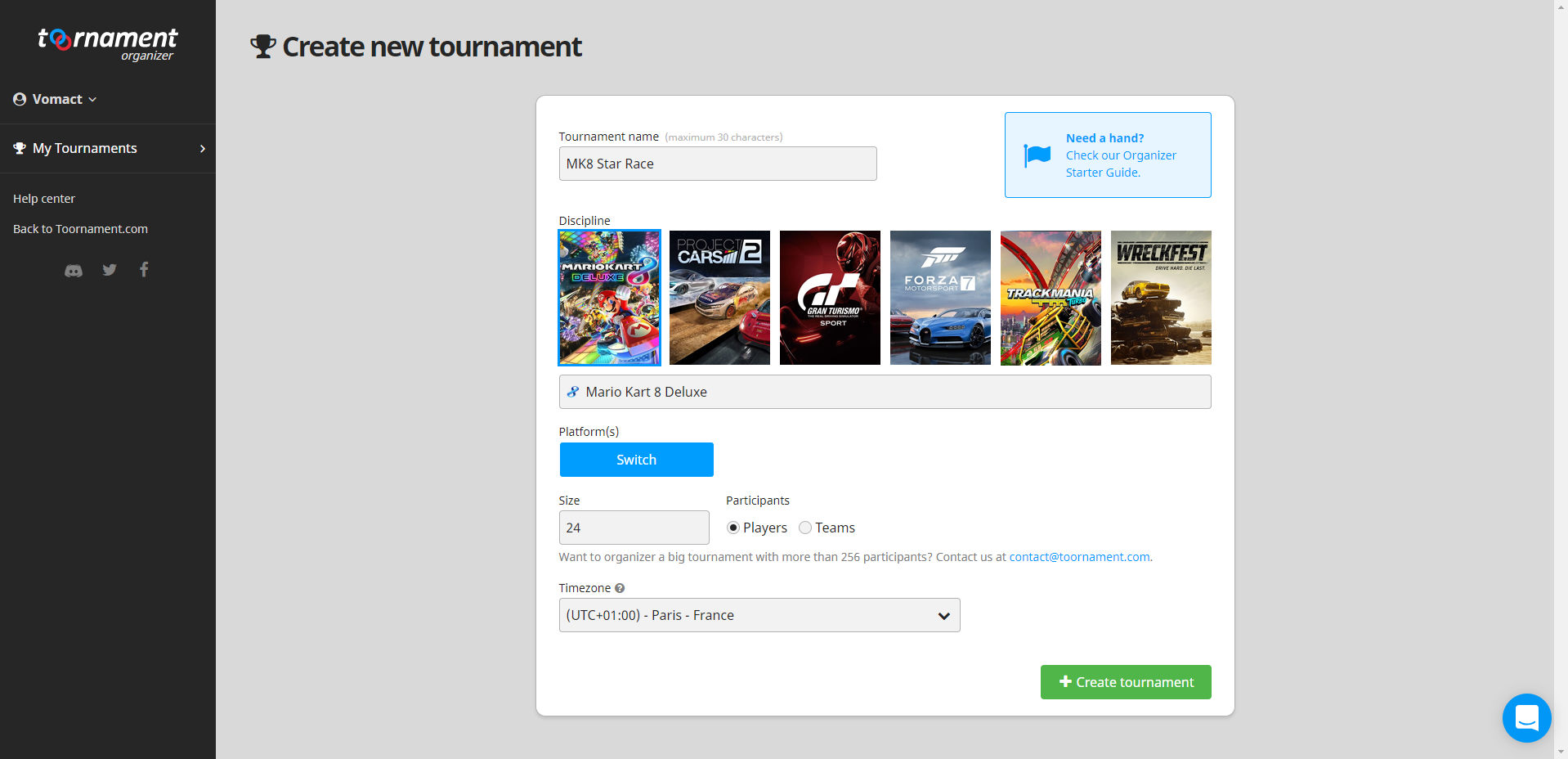In the image, we observe a computer dashboard designed for organizing tournaments. On the left side of the screen, there is a dark gray sidebar featuring a section titled "Tournament Organizer," distinguished by an icon that comprises two overlapping circles—one red and one blue. The username "vomcat" is displayed here as a drop-down option. Additional options in this sidebar include "My Tournaments" with a small trophy icon next to it, as well as links to the "Help Center" and "backtotournament.com." Beneath these, there are icons representing social media links for Discord, Twitter, and Facebook.

The main portion of the screen, which has a lighter gray background, includes a central large gray box labeled "Create a New Tournament." Within this box is a smaller white box where you can input the "Tournament Name." There is a section labeled "Discipline" that lists five different video games for selection. Upon choosing a game, the name of the selected video game is displayed. Further options available in the white box allow you to choose your platform, specify the size and number of players or teams, and select your time zone. Below these options, there is a button to "Create Tournament."

In the top corner of this white box, there is a small blue box that prompts, "Need a hand? Check out our organizer starter guide," accompanied by a blue flag icon. At the very bottom of the entire screen, a small blue chat icon is visible, which appears to offer support-related assistance.